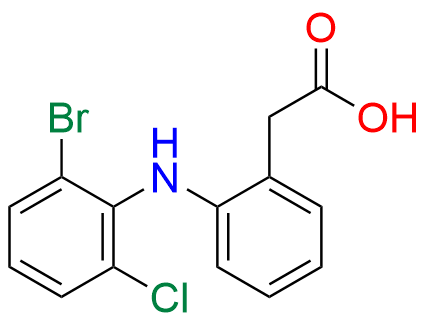The image features a scientific diagram of molecules on a white background. The primary structures are two hexagonal molecules, illustrated with black lines. On the left, the first hexagon is labeled "Br" in green. Connected to it by two lines, the lower line bears the label "Ci" in green, and the upper line connects to "Hn" in blue. The "Hn" label leads to the second hexagon in the diagram. From the top of this second hexagon, an additional line extends upward and branches out, forming a partial hexagonal shape. At the top of this branch is the label "O" in red, and along its right side, there are the letters "OH," also in red. This detailed depiction emphasizes the connectivity and layout of the molecules.